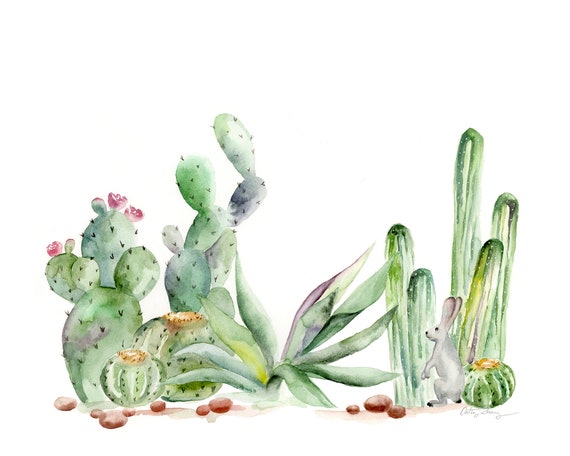This landscape-format illustration in color portrays an arid desert scene brimming with a variety of cacti and desert elements. Prominently on the right-hand side, a gray-furred rabbit with notably long ears peers curiously toward the center of the image. The desert floor, represented by a strip of dirt, is interspersed with brown rocks of various sizes.

On the left, the scene features an array of cacti, including prickly pear cacti adorned with blue and pink blossoms. Other cacti types such as organ pipe-like or young saguaro cacti stand tall, particularly near the rabbit. Additional cacti include the round-brain type and some that resemble green pumpkins in their peculiar shapes. The painting, rendered in watercolor, highlights the textures and shades of green in the various cactus species, some round and puffy with visible spikes, while others are tall and smooth. The backdrop is a pristine white, accentuating the vibrant flora and reinforcing the arid, minimalist desert ambiance.